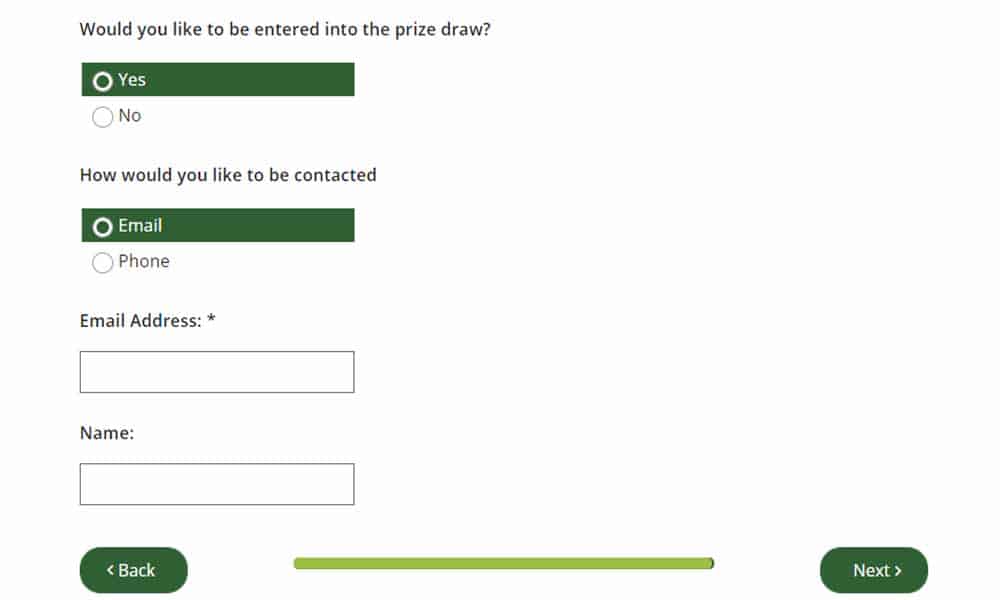The screenshot depicts a webpage designed for entering information for a prize drawing. The page features a clean, white background with black text. At the top, it poses the question, "Would you like to be entered into the prize draw?" Beneath this question are two selection buttons: a wide, rectangular, dark green button for "Yes," which is highlighted and currently selected, and an option for "No."

Following this, another section titled "How would you like to be contacted?" appears in black text. Below this, there are options for either email or phone contact. The "Email" option is selected, also displayed on a wide, rectangular, dark green bar.

Additional fields for user input are located below these selection areas. The first input field, marked with an asterisk, is intended for an email address and is currently blank. The second input field, also blank, is for the user's name.

At the bottom of the form are two navigational buttons. On the left side, an oval, dark green button labeled "Back" is accompanied by a backward arrow. On the right side, a similar dark green button labeled "Next" features a forward arrow. These two buttons are separated by a wide, light green line. The design emphasizes ease of use with clear instructions and a straightforward layout.